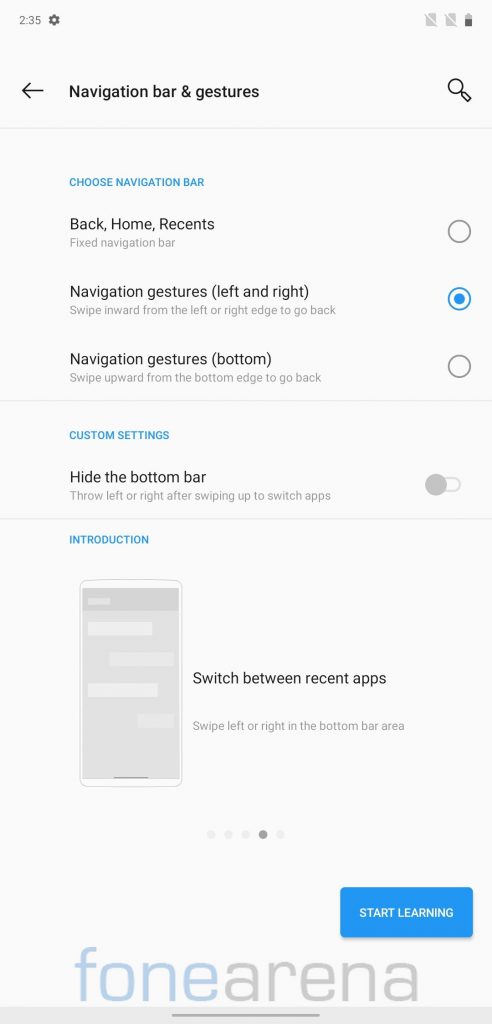**Detailed Caption:**

This image is a screenshot of the "Navigation Bar and Gestures" settings on a mobile phone. The title "Navigation Bar and Gestures" is prominently displayed at the top of the screen, with a magnifying glass icon to its right, indicating a search functionality.

The settings window is divided into three distinct sections:

1. **Choose Navigation Bar**:
   - This section allows users to select their preferred navigation style. 
   - The section title "Choose Navigation Bar" is highlighted in blue, and the options beneath it are in black text. 
   - There are three navigation options listed:
     - "Back, Home, and Recent"
     - "Navigation Gesture - Left and Right" (this option is currently selected, indicated by a filled bubble next to it)
     - "Navigation Gesture - Bottom"

2. **Custom Settings**:
   - The custom settings section, also with a blue title, features a single toggle option.
   - The option "Hide the bottom bar" is displayed here, but it is not toggled on.

3. **Introduction**:
   - This instructional section is marked with a blue title and contains a sketch of a mobile phone to illustrate its point.
   - To the right of the sketch, there are instructions: "Switch between recent apps. Swipe left or right in the bottom bar area."
   - At the bottom right corner of this section, there is a blue "Start Learning" button for initiating a learning process about the gestures.

At the very bottom of the screen, in the center, is the name "phone arena," styled uniquely with "phone" in blue (starting with a lowercase 'f') and "arena" in gray, all in lowercase and merged into one word.

The overall background of the settings window is white, giving the entire screen a clean and organized appearance.